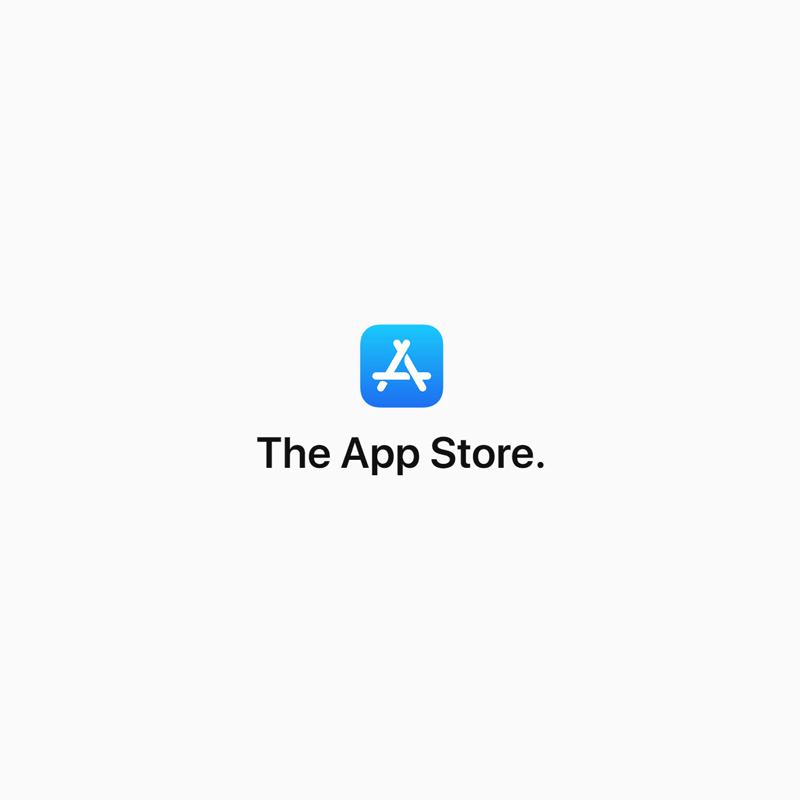The image features the iconic logo of the Apple App Store set against an eggshell white background. Centrally positioned, the App Store icon is a square with rounded edges showcasing a blue gradient that transitions from a darker shade at the bottom to a lighter blue at the top. Dominating the center of the icon is a stylized 'A' composed of three white stick-like elements resembling tongue depressors. Directly beneath this logo, the words "The App Store." are displayed in bold, black font, with each word starting with a capital letter: "The" with a capital T, "App" with a capital A, and "Store" with a capital S.